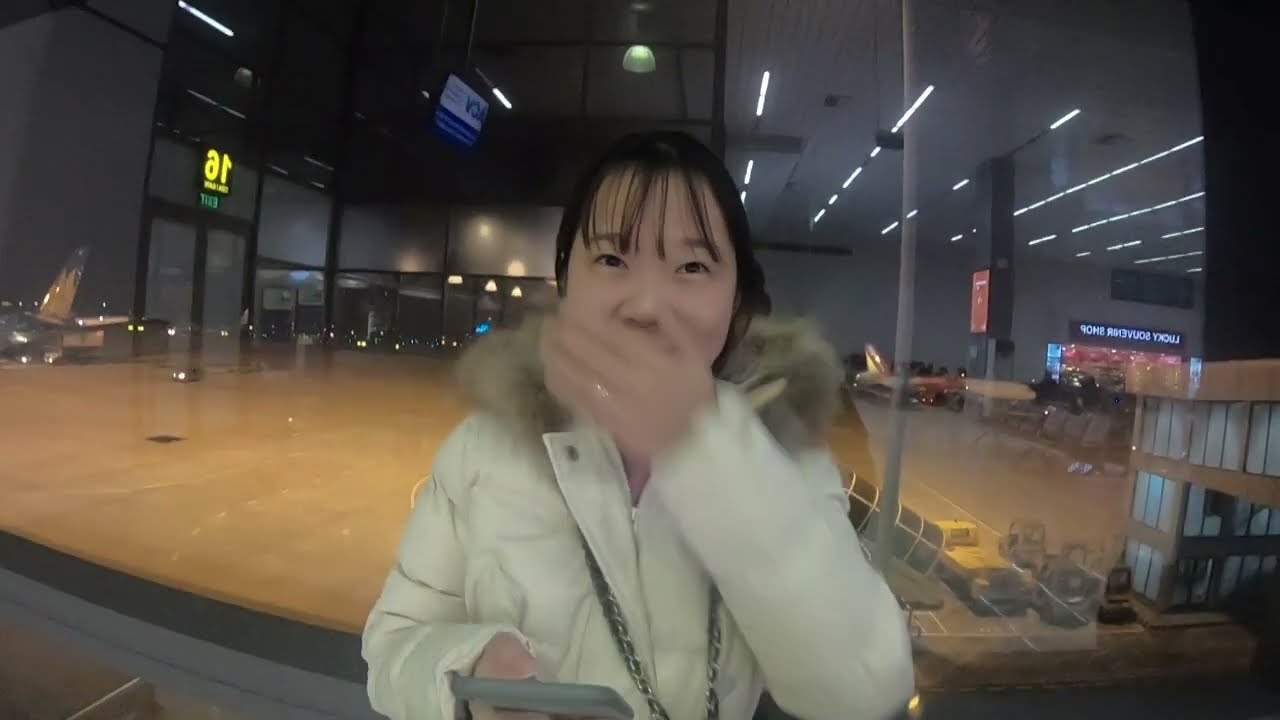This photograph features a young Asian woman, likely in her late 20s, with short, straight black hair and bangs. She is captured mid-laugh, coyly covering her mouth with her left hand, which appears slightly blurry due to motion. Her right hand, bent at the elbow, holds a cell phone. She is wearing a puffy white jacket with a beige fur-lined hood, left unzipped to suggest she is indoors.

The background reveals she is in an airport terminal. Large glass panes behind her expose a view of parked cars, airport vehicles, and airplanes lined up at gates. Reflections of shop signs, including letters such as "A1," are visible on the glass. The floor of the terminal is brown, and additional details like a lanyard or necklace around her neck and a ring on her ring finger further enrich the scene. This comprehensive description captures the essence and context of the image, emphasizing the shared and repeated observations from all four captions.